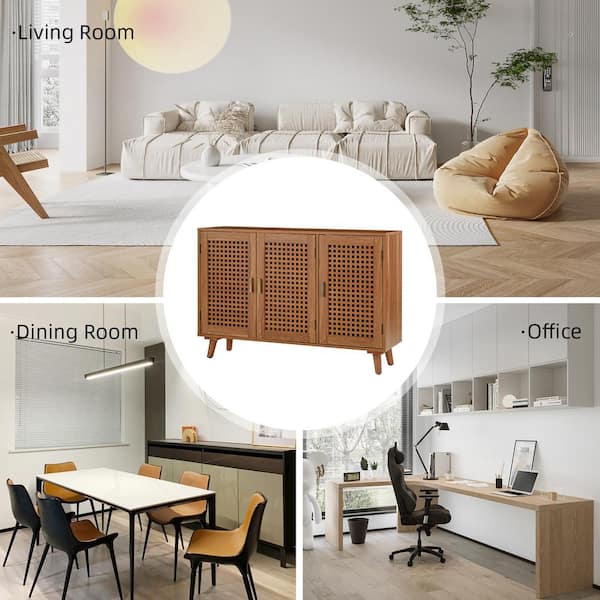This detailed photograph is a square-shaped composite advertisement, divided into an upper half and a lower half. The top half features a single, labeled photograph of a "Living Room." This section reveals a cozy, white-themed living room with a fluffy white sofa, a large square white rug, and a beige wooden floor with chevron patterns. Adjacent to the sofa, on the right, is a cream-colored beanbag and a lush tree-like plant. Behind these furnishings, a white wall holds an image of a shining, light-yellow sun.

The lower half of the composite is split into two equal sections. To the left, we find the "Dining Room," showcasing a long rectangular white table surrounded by six chairs that are black on the outside and brown on the inside. White walls encompass this area, and closed blinds can be seen on the left side of the room. On the right side of the lower half, the "Office" is featured. This room has gray walls with shelving, a light brown wooden floor, and a spacious L-shaped light brown desk. A black computer chair faces the desk, with a window to the left and a black garbage can on the floor.

Prominently centered within the entire image is a circular photograph of a distinctive brown wooden cabinet with three doors, each featuring lattice work, standing on four small legs. This unique piece is not visible in any of the individual room images but is highlighted separately due to its decorative appeal.